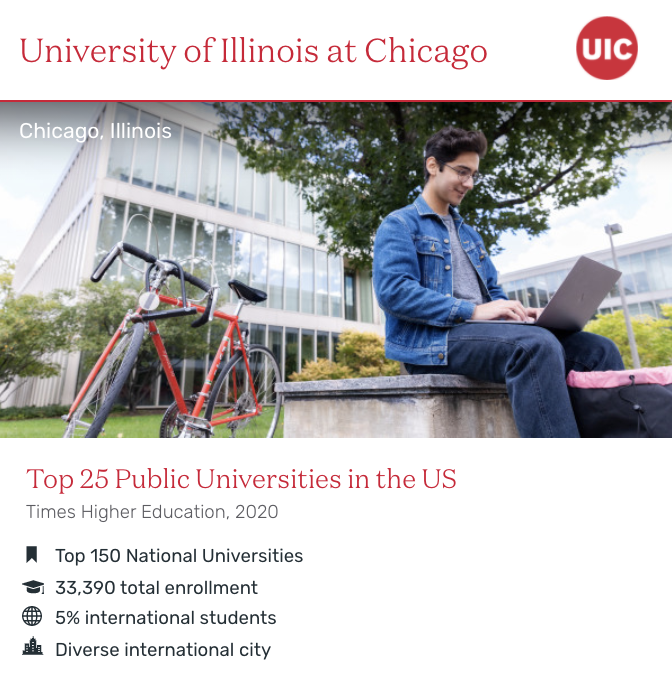### University of Illinois at Chicago Website Banner Description

At the top of the webpage, the text "University of Illinois at Chicago" is prominently displayed in bold red letters. Below this, a red circle featuring the letters "UIC" in white is situated. Beneath the UIC emblem, an image announces "Chicago, Illinois" in white text located in the upper left corner. 

The central image portrays a serene moment on campus, illustrating a young man sitting on a concrete bench. The student, clad in jeans and a gray shirt layered under a denim jacket, balances a laptop on his lap. He has dark hair, wears glasses, and appears deeply engaged in his work. A tree and several campus buildings, characterized by their modern glass exteriors and three-story structures, form the background, creating a scenic and academic atmosphere.

Adjacent to where he is seated, a red bicycle is parked, adding a splash of color and vibrancy to the setting. At his feet, a backpack rests casually on the ground, indicating his preparedness and active student life.

Towards the bottom of the image, there are several informational statistics:
- "Top 25 Public Universities in the U.S." – Times Higher Education 2020
- "Top 150 National Universities"
- "33,900 Total Enrollment"
- "5% International Students"

This detailed portrayal not only highlights the university's vibrant campus life but also its esteemed academic standing and diverse student body.